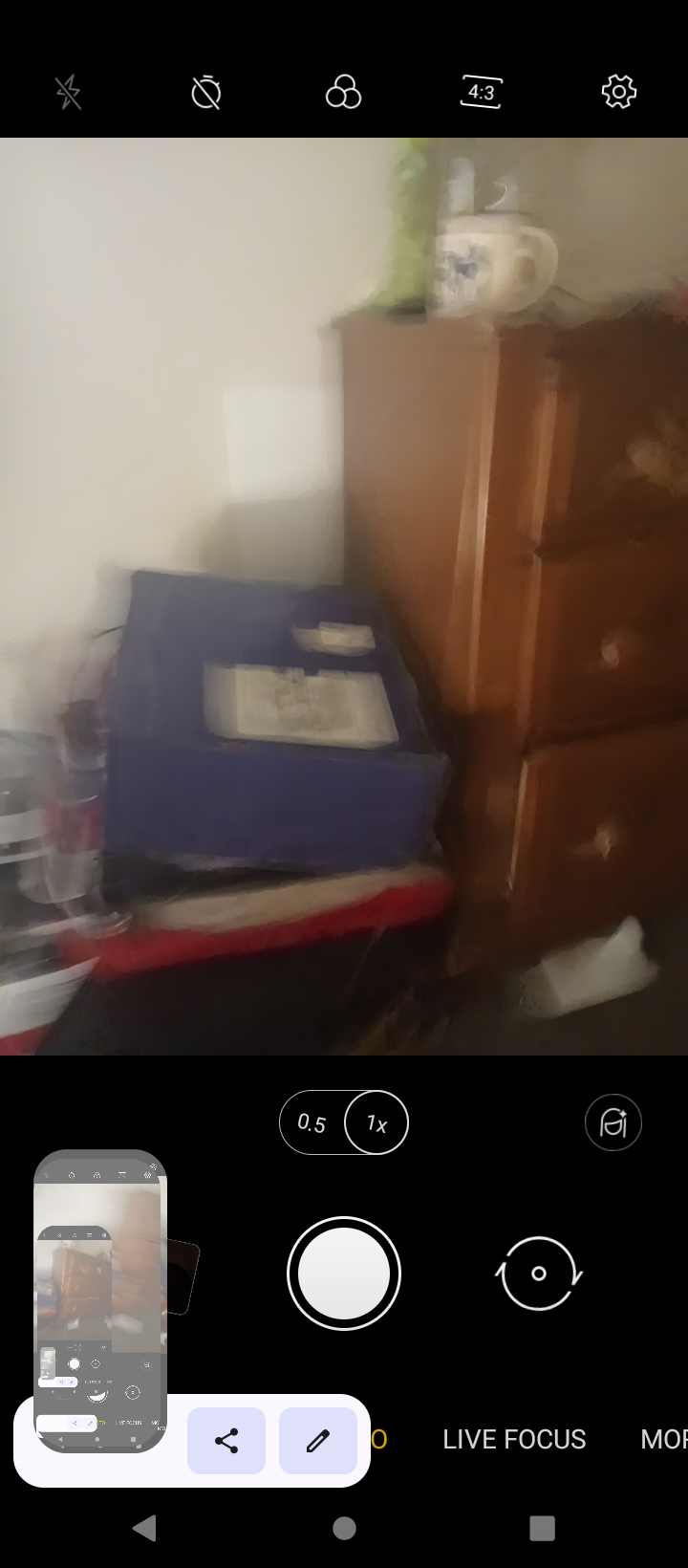This screenshot captures a phone's camera interface in picture-taking mode. The scene displayed is slightly blurry, making some elements difficult to discern clearly. On the right side of the image, there is a partial view of a bureau with three drawers. Resting on top of the bureau is a white coffee cup adorned with a blue design, containing some indistinguishable items sticking out of it. To the left of the bureau, there is a blue box with a mailing label affixed to its top, sitting on a small table covered with a striped cloth. On the bottom part of the screen, the photo button is visible, and a miniaturized version of the phone screen is shown on the lower-left side. The photo settings indicate a 1x zoom, and the "Live Focus" mode is active, as noted on the bottom right of the screen.